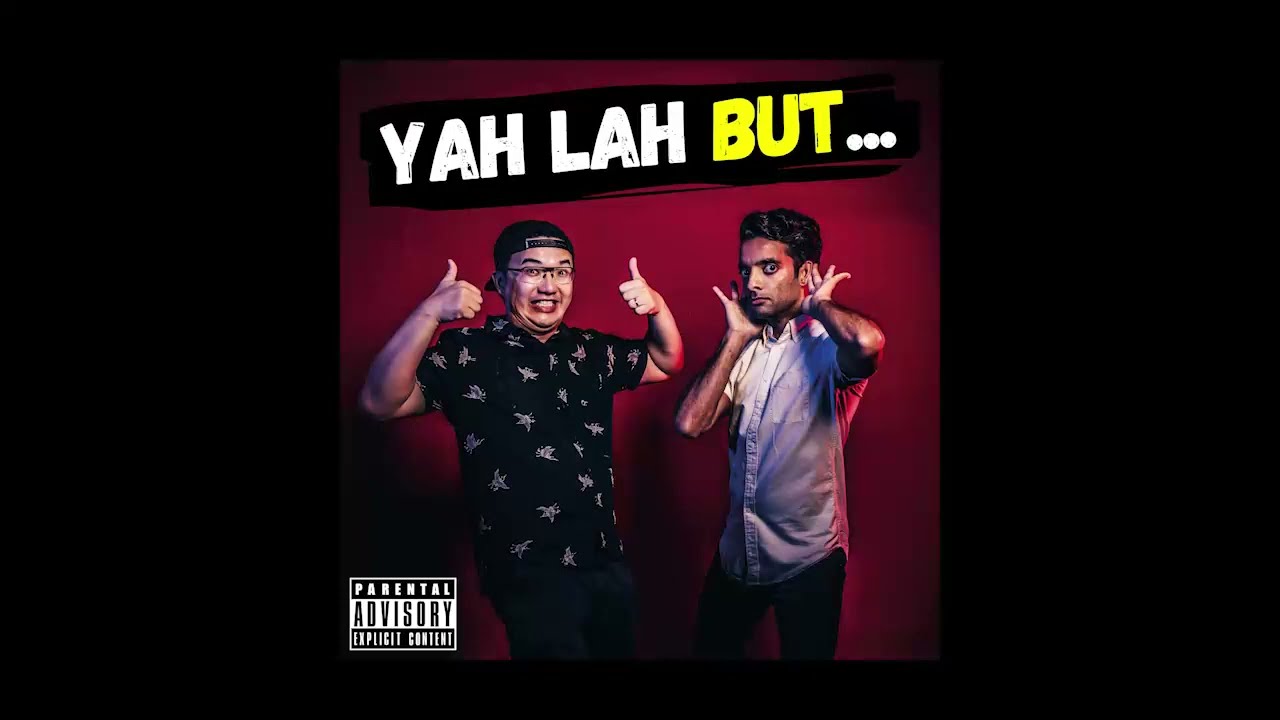The image appears to be album artwork featuring the title "Ya Lah But..." at the top. The text "Y-A-H-L-A-H..." is displayed, with "Ya" and "Lah" in white and "But..." in yellow. The background is a rich maroon or magenta color. In the foreground, there are two men. 

The man on the left, who seems to be East Asian, sports a backwards black cap and glasses and is dressed in a black shirt with a white design and jeans. He is enthusiastically giving a thumbs up with both hands and smiling. To his right is a man who appears to be South Asian, with black hair, wearing a white button-up shirt and black jeans. He looks engaged and has his hands cupped around his ears, as if trying to hear something.

A "Parental Advisory, Explicit Content" label is present in the bottom left corner. The background includes a black brushstroke at the top, serving as the backdrop for the album title. Overall, the image captures a lively moment between the two men against a vibrant backdrop, indicative of the dynamic content their album might contain.